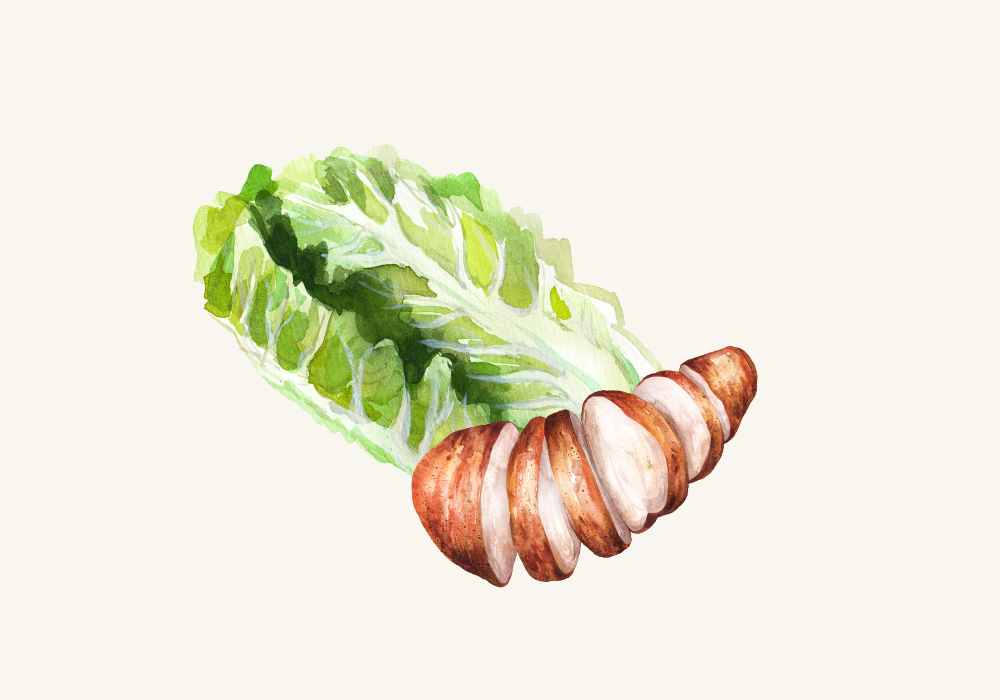The image is a delicate watercolor painting featuring a russet potato and romaine lettuce, set against a plain white background. The potato, brown on the outside and white on the inside, is sliced into six pieces and displayed in a slightly fanned-out arrangement towards the bottom right. The large, light green romaine lettuce leaves, tinged with paler green stems and darker green where the stalks converge, rise above the potato, creating a layered effect. The overall composition uses soft, wispy watercolor techniques, with the potato and lettuce taking up about 40% of the space in the otherwise stark, grayish-white background. The lack of text or additional detail emphasizes the simple, serene nature of the scene.